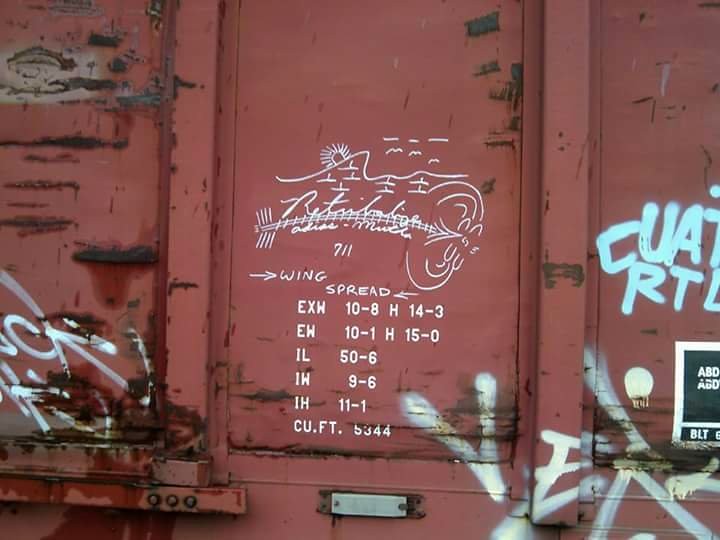The image captures a close-up of a weathered metal wall, likely the side of a train car or shipping container. The metal surface is aged, with patches of rust and chipped paint revealing its prolonged exposure to the elements. Prominent graffiti in shades of light blue and white can be seen, with the white graffiti concentrated at the bottom right and blue graffiti to its side. At the center of the wall, a white, script-like graphic depicts a mountain, a sun, and possibly train tracks, alongside the words "wing spread," followed by several acronyms such as EXW, EW, IL, IW, IH, accompanied by numerical values. The bottom row contains the more familiar term "cubic feet," specifying the volume as 5344. Additional markings and some black spots are scattered across the upper and lower corners. A silver rectangular handle is visible at the bottom part of the wall, further suggesting this is the side of a rail car.